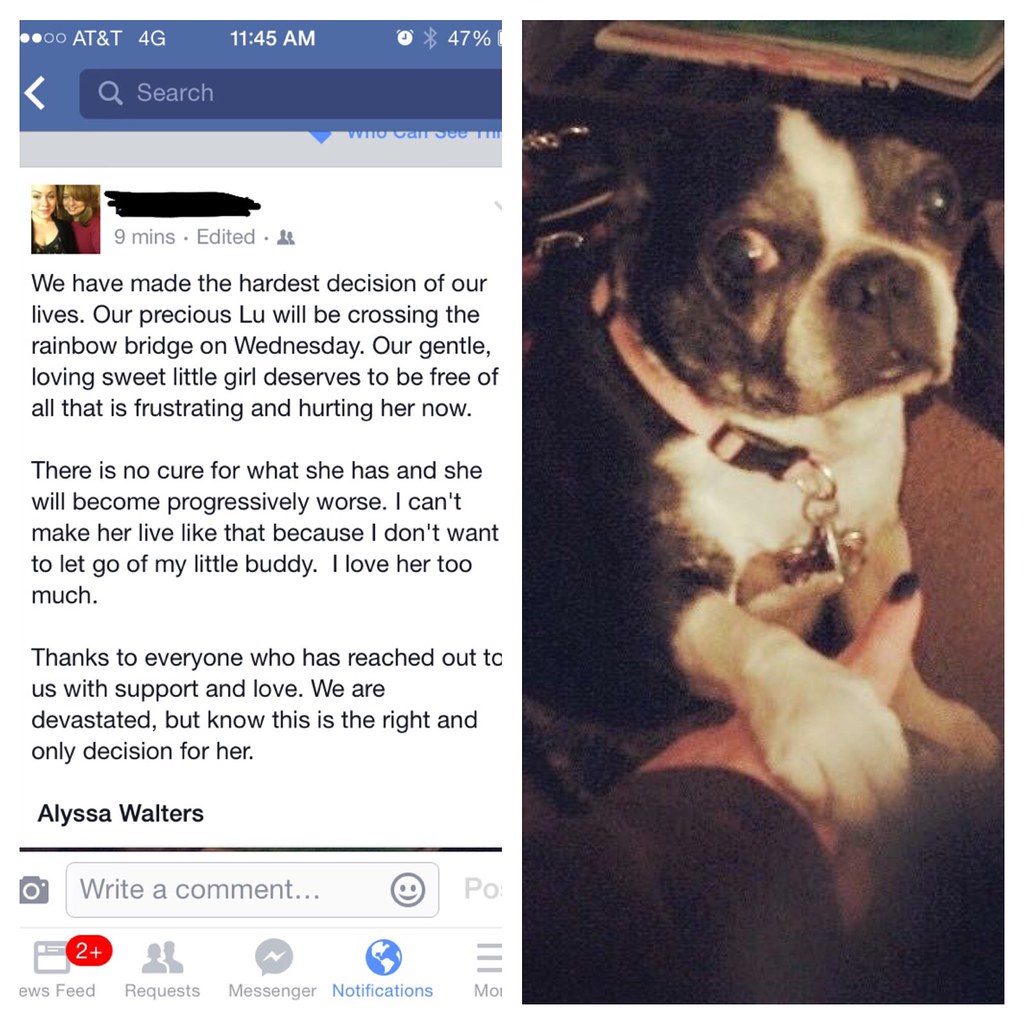In this emotionally charged image, we see a screenshot from an iPhone's Facebook application, captured at 11:45 AM on an AT&T network with the battery at 47%. On the left side of the screen, a heartfelt post by Alyssa Walters is displayed, detailing their agonizing decision to euthanize their beloved dog, Lou, who is suffering from an incurable and progressively worsening condition. Alyssa expresses deep gratitude to those who have offered support, acknowledging the devastating but necessary choice to let Lou, described as a gentle and loving companion, "cross the Rainbow Bridge."

The post is accompanied by a poignant photograph on the right side of the screen, showing little Lou, a black and white bulldog, looking directly at the camera with sad eyes. Lou's paw rests on a person's hand, symbolizing the strong bond and affection they share. The image is cast in tones of black, white, red, blue, gray, and brown, reinforcing the somber mood of the message.